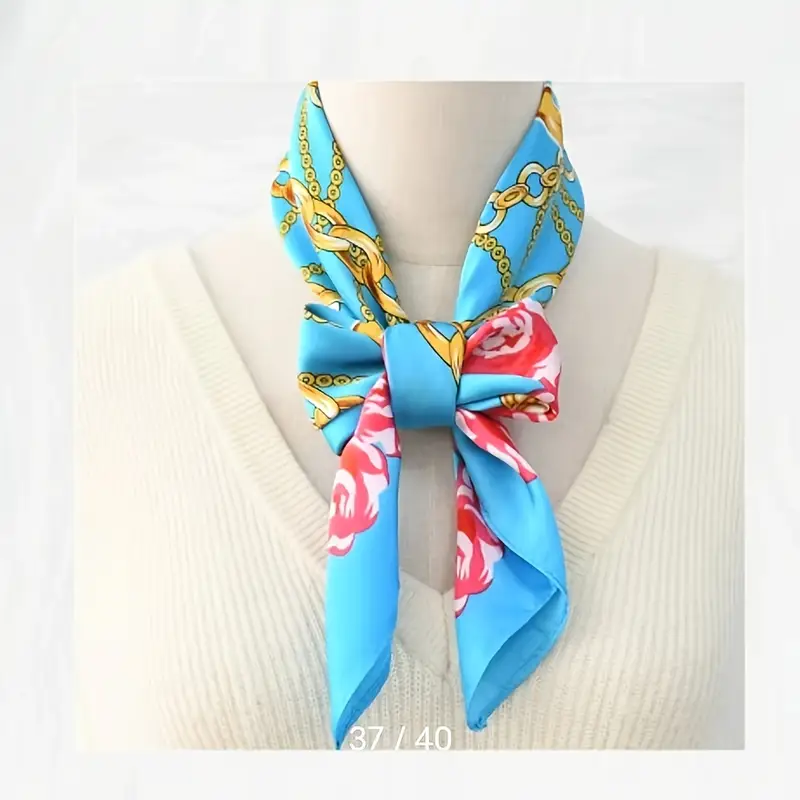The image showcases a white mannequin against a white background, indoor setting, adorned with a vibrant ensemble. The mannequin is attired in a white v-neck sweater featuring a ribbed pattern along the collar and diagonally set gold accents, enhancing the texture. Draped around the neck is a blue and red floral print scarf embellished with intricate gold chain designs. The scarf is elegantly tied into a bow, displaying a playful array of dark pink, almost red, and light pink petals amidst its rich blue background and golden links. Notably, at the bottom of this meticulously styled image, white text reads "37/40," potentially indicating a size or series number. The lighting source from the left accentuates the contours of the mannequin, capturing the subtle yet detailed aesthetics of the outfit.